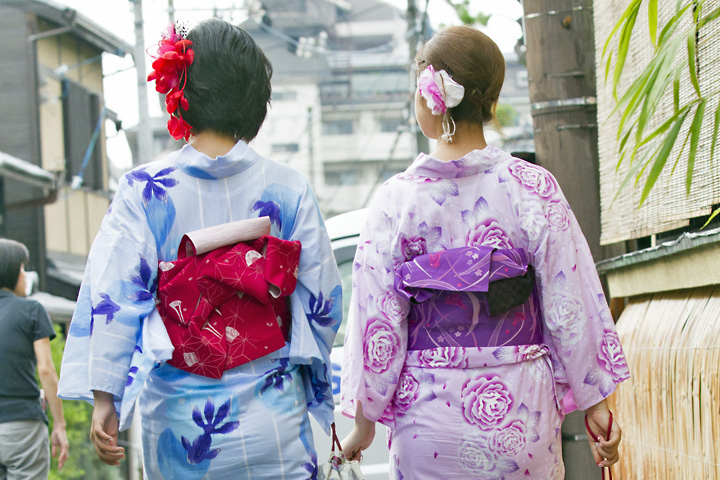The photograph captures two women, viewed from behind, walking down the street during the day. The woman on the left is wearing a light blue Asian-style robe adorned with dark blue flowers, and a bright red belt featuring a star pattern. She has short black hair, complemented by a striking red flower pinned near her left ear. The woman on the right sports a light and dark purple Asian-style robe with dark purple rose patterns, along with a bright purple belt decorated with a swishy pattern. Her short brown hair is neatly tucked back, and she has a white and purple flower pinned on the left side. Both women walk side by side, amidst an urban landscape with tall buildings in the distance. Bamboo flanks the right side of the image, while additional buildings are visible in the background. A person in a black t-shirt, cap, and pants, with their arm outstretched, is also seen in the vicinity.